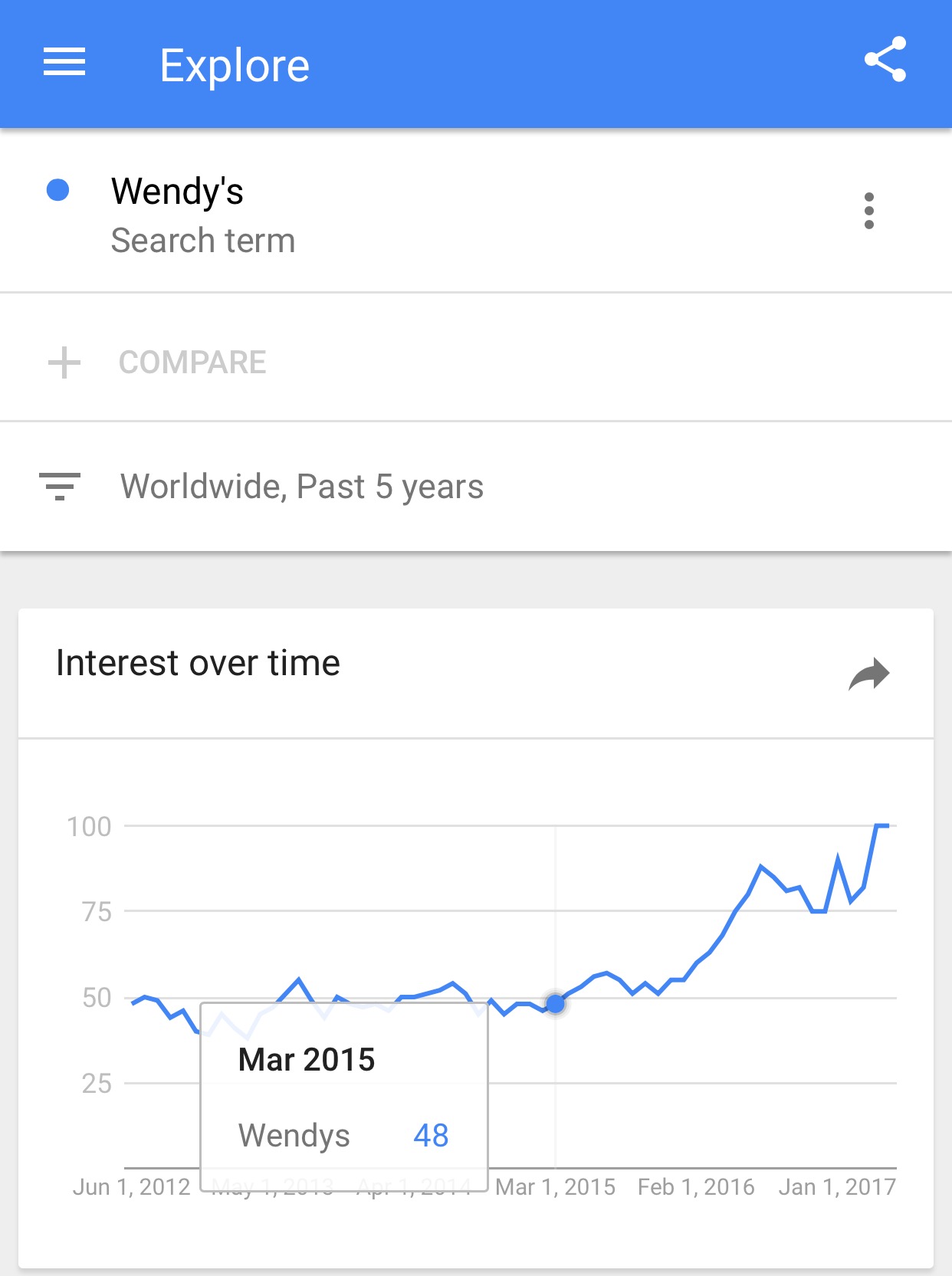This image is a detailed screenshot from a website or app interface. At the top, a blue navigation bar spans the full width, featuring white text. On the left side of this bar, there is a hamburger menu icon followed by the word "Explore." On the right side, the share button is represented by a triangle with dots at each vertex.

Beneath the blue bar, aligned to the left, a small blue dot is followed by the bold text "Wendy's," with the phrase "search term" written in gray beneath it. To the right, three vertical dots indicate a dropdown menu, and below this, a grayed-out plus sign accompanied by the word "Compare."

Further down, there is a filter or sort icon, next to which the text "Worldwide, past five years" is displayed. At the bottom segment of the screenshot, a line graph is presented, entitled "Interest over time." To the right of the graph's title is an arrow icon, another share feature.

The graph itself is rendered in blue and tracks interest over a timeline. The vertical axis is marked at intervals of 25, ranging from 0 to 100. The horizontal axis is labeled with specific dates: June 1, 2012; May 1, 2013; April 1, 2014; March 1, 2015; February 1, 2016; and January 1, 2017. A specific data point is highlighted at March 2015, showing an interest value of 48 for "Wendy's."